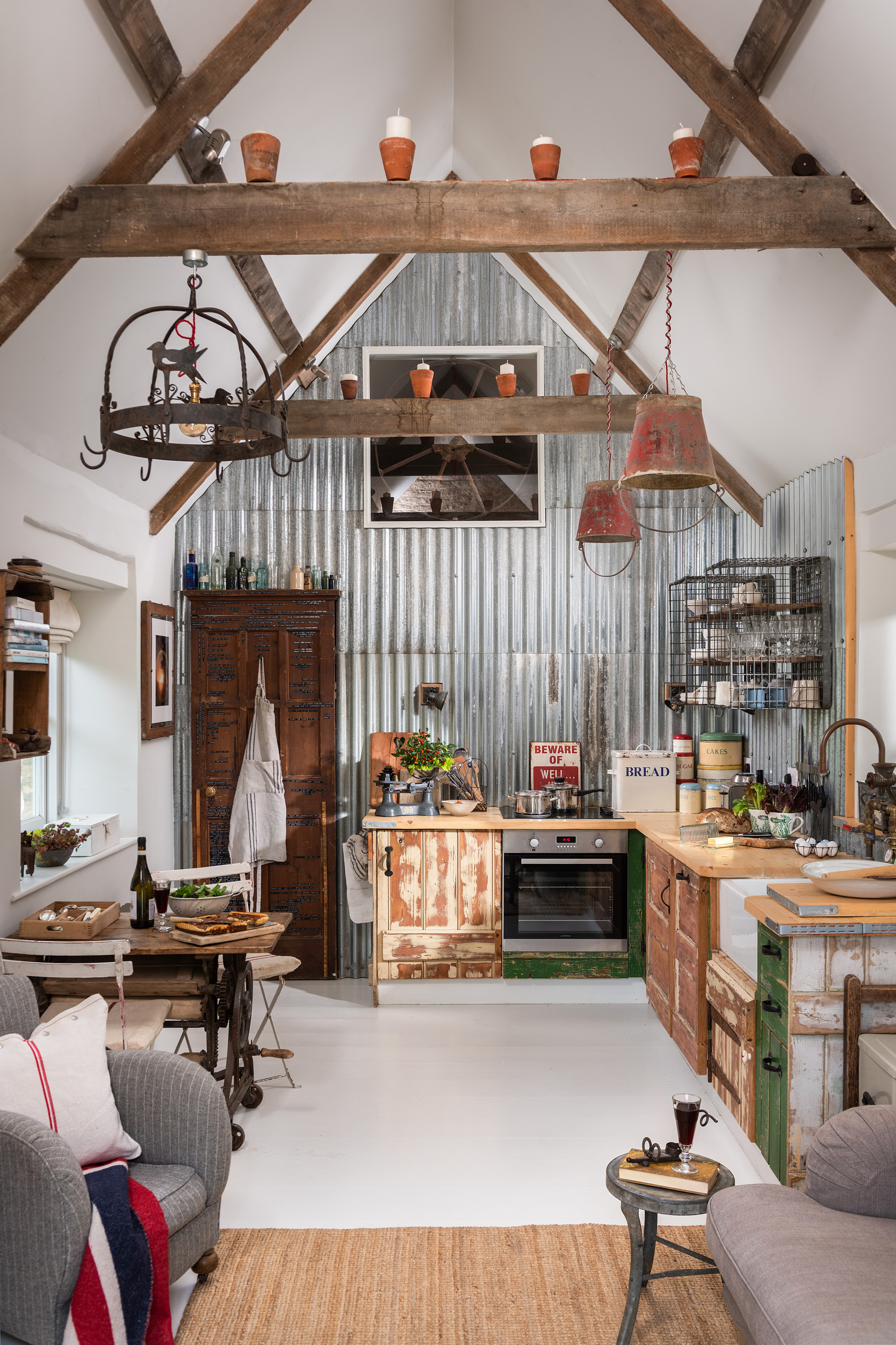This color photograph captures the interior of a tiny house or cabin, meticulously fashioned using upcycled and repurposed materials. The scene faces the end wall of the kitchen, which is lined with decorative aluminum siding or wavy tin sheets, giving it a rustic charm. The mismatched kitchen cabinets show signs of wear, suggesting their second-hand origins. Above the sink area, cups are stored in a creative shelving unit made from a metal wire cage, turned on its side. A modern electric cooktop contrasts with the assorted wooden cabinet doors. Antique lanterns hang in the space, with two lights ingeniously crafted from upside-down metal buckets, repurposed feed buckets with holes drilled and wired for electrics. The room is adorned with numerous little bottles and country-style knickknacks, enhancing its quaint, eclectic feel. The furniture, including a sofa and chair at the bottom of the image, appears clean and new. The floor features a blend of wood or perhaps a rug and white tiles in the kitchen area. The overall aesthetic is one of innovative reuse within a cozy, upcycled living environment.